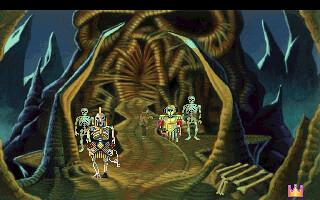The image is a detailed still from a game, showing a small rectangular scene set in an intricately designed cave. The interior is predominantly brown, with shades of gold and black forming a pathway that leads into the depth of the cave. On the left side, there is a brightly colored white skeleton standing next to another skeleton figure adorned in gold armor and a matching gold mask. In front of this figure is another character dressed in yellow armor, accented with pink, also wearing a mask. Surrounding these figures are various other colored skeletons: one in yellow and red, another in pinkish tones resembling a dog, a whitish-green one, and another with hints of blue and pink. The cave also features thin, curved mountains, possibly rendered in a surrealistic style, with pointy tops visible in the background. Outside the cave, there is some sort of bench or stairs and brown evergreen trees. In the right corner, a small pink crown with a gold centerpiece is prominently displayed, adding a touch of regal elegance to the otherwise eerie scene.